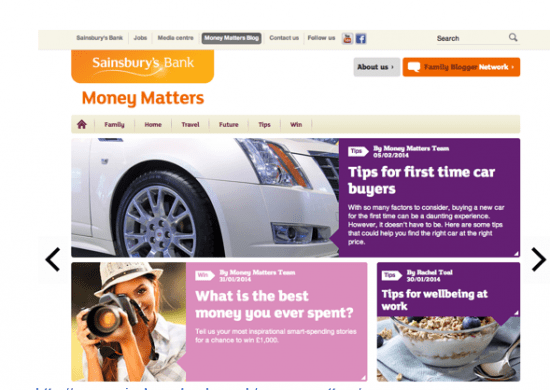The image depicts a bank login page for Sainsbury's Bank. At the top of the page is a menu bar, divided into several sections. In the upper left corner, it reads "Sainsbury's Bank". Progressing to the right, there are tabs labeled "Jobs", "Media Center", and the highlighted tab "Money Matters Blog". Continuing to the right, there are the "Contact Us" and "Follow Us" sections, the latter featuring YouTube and Facebook logos. The far right of the menu bar contains a search box with the placeholder text "search" and an adjacent magnifying glass icon.

Just below the menu bar, there is another Sainsbury's Bank logo in orange, positioned in the upper left, with the words "Money Matters" displayed beneath it, also in orange. To the right of this logo and text is a tab titled "About Us", followed by an orange and white icon labeled "Family Blogger Network", which also features some bronze lettering.

Directly below "Money Matters", there's an additional set of menu items featuring icons and text for various categories. These include, from left to right: "Home", "Family", "Home" (again), "Travel", "Future", "Tips", and "Win".

Further down the page, the content shifts to showcasing articles. The first article features an image of a white car, displaying the front right section and the front right wheel. To the right of this image, there is text on a purple background that reads "Tips for First-Time Car Buyers", indicating an article subheading.

Below this section are two more article previews. The left section shows an image of a woman holding a camera and smiling slightly. Adjacent to this image, the text reads "What is the Best Money You've Ever Spent?”. To the right of this, another box displays "Tips for Well-Being at Work" beside an image of a bowl filled with granola, berries, and yogurt.